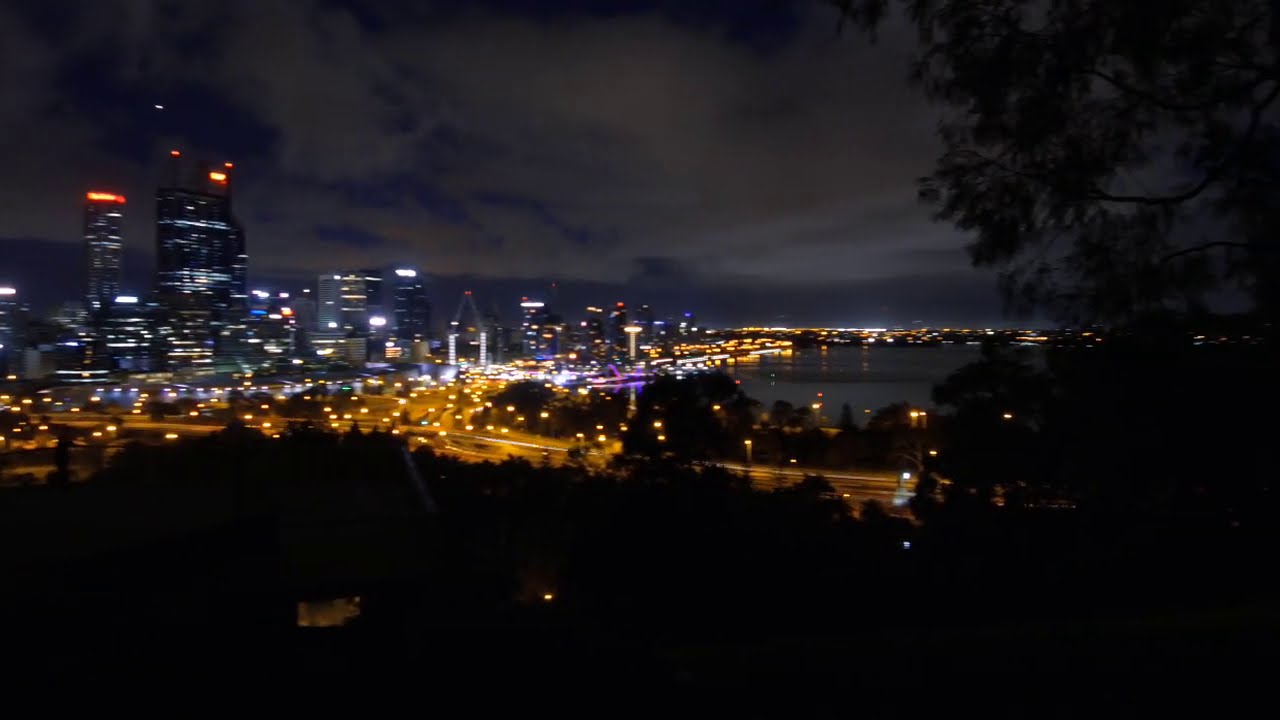The image captures a bustling city skyline at night, illuminated by a myriad of lights. The road entering the city from the right is accentuated by a thickening stream of yellow streetlights leading towards the center. As the road merges with the city, the yellow lights diverge left and upwards in the image. The left side of the cityscape is dominated by towering skyscrapers adorned with varying hues of blue lights and capped with striking orange lights. Tall buildings scatter the landscape, contributing to the lively city atmosphere. 

In the upper right corner, the silhouette of a thick tree is visible, adding a touch of nature to the urban scene. In the distance, a sizeable body of calm, almost black water borders the edge of the city, reflecting the tranquility of the night. The very bottom of the image, beneath the highway, is completely dark save for a single speck of light. The sky above is heavily clouded, with only slivers of very dark blue peeking through, indicating a recent sunset and a thick cloud cover. The foreground features a mix of foliage and yellow streetlights, tying the scene together as a quintessentially busy yet serene nighttime cityscape.